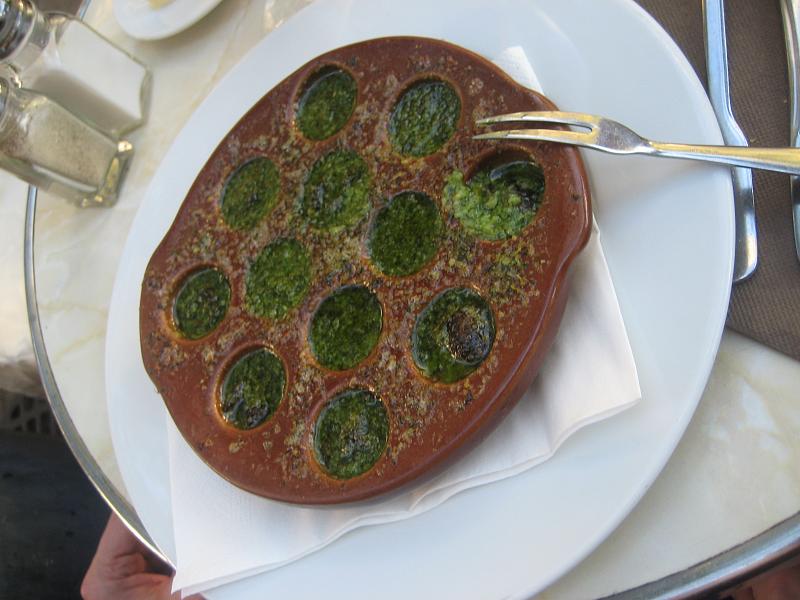In the image, a brownish-red escargot serving dish with 12 circular indentations, each filled with a dark mossy green sauce, is centered on a white napkin that itself rests on a larger round white china plate. The dish, which may also be used for oysters Rockefeller, is the main focus. A two-pronged fork is placed horizontally on the right side of the serving dish. The table beneath is made of a white or cream-colored marble or alabaster material. In the top left corner of the image, partially cropped out, is a salt and pepper shaker. At the bottom left, a part of someone's hand is visible, hinting at a dining setting.